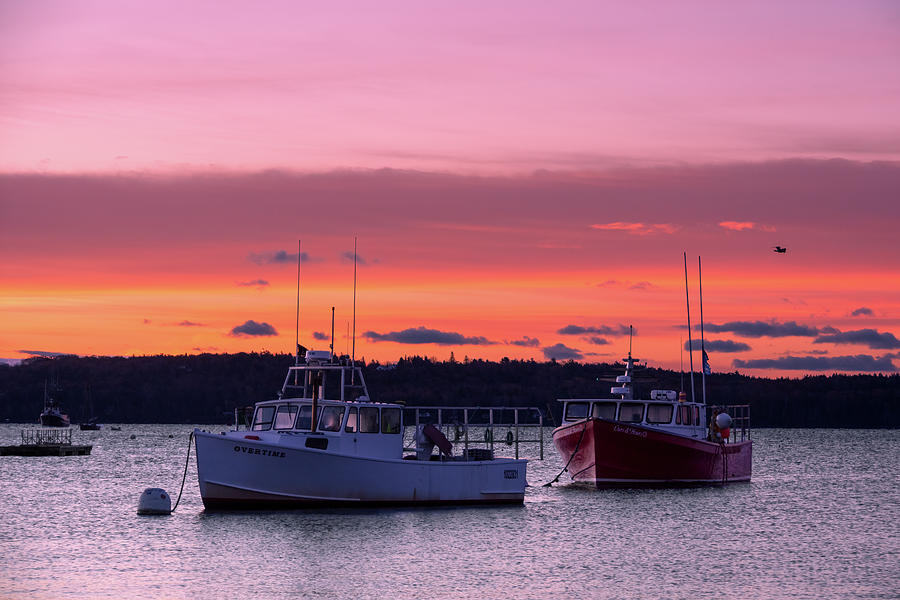The photograph depicts a serene harbor at sunset, with a rich palette of pink, yellow, orange, and red hues accentuating the sky. The foreground features two boats adrift in dark blue waters. The foremost boat, a white vessel named "Overtime," bears noticeable rust towards its lower section and has several windows on its upper structure. Just behind it, a dark red boat with indistinguishable white lettering and multiple upper windows contrasts against the water. Both boats appear to be tethered, possibly to buoys, suggesting they are stationary. A dock can be seen to the left of these boats, and several other boats are faintly visible in the background. Bordering the harbor are lush dark green trees, adding a natural enclosure to the scene. Additionally, either a bird or a plane is faintly discernible in the sky. The overall ambiance of the photo conveys tranquility and beauty, making it an inviting day for maritime activities.